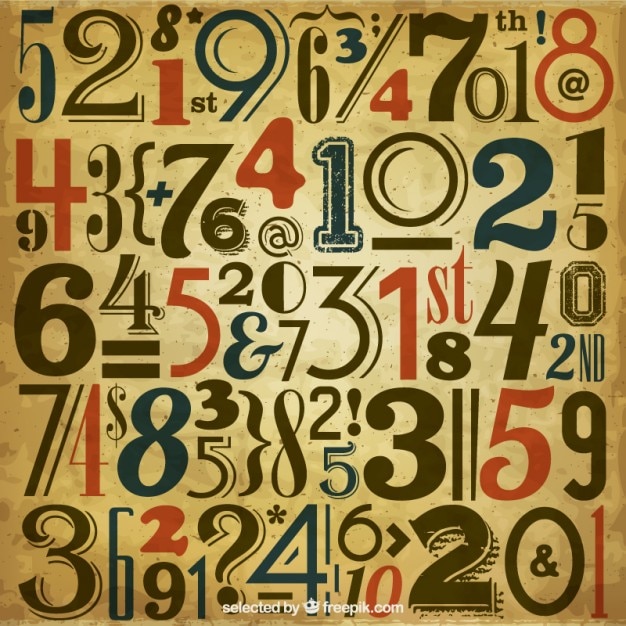This photograph features a decorative design on an off-yellow or tan background that looks somewhat weathered or like old gift wrap paper. The design consists of a random assortment of numbers and symbols displayed in a variety of unique fonts and colors—primarily dark red, dark brown, and dark blue. Numbers from 0 through 9 are scattered across the image, with additional text elements like "first," "seventh," and "second." Symbols such as exclamation points, question marks, asterisks, plus signs, dollar signs, and parentheses are interspersed among the numbers, contributing to the chaotic yet intriguing pattern. The bottom of the image features a white text that reads "Selected by FreePic.com" along with an accompanying logo of a white crown. This visually engaging poster could be used for educational or decorative purposes, potentially related to mathematics.